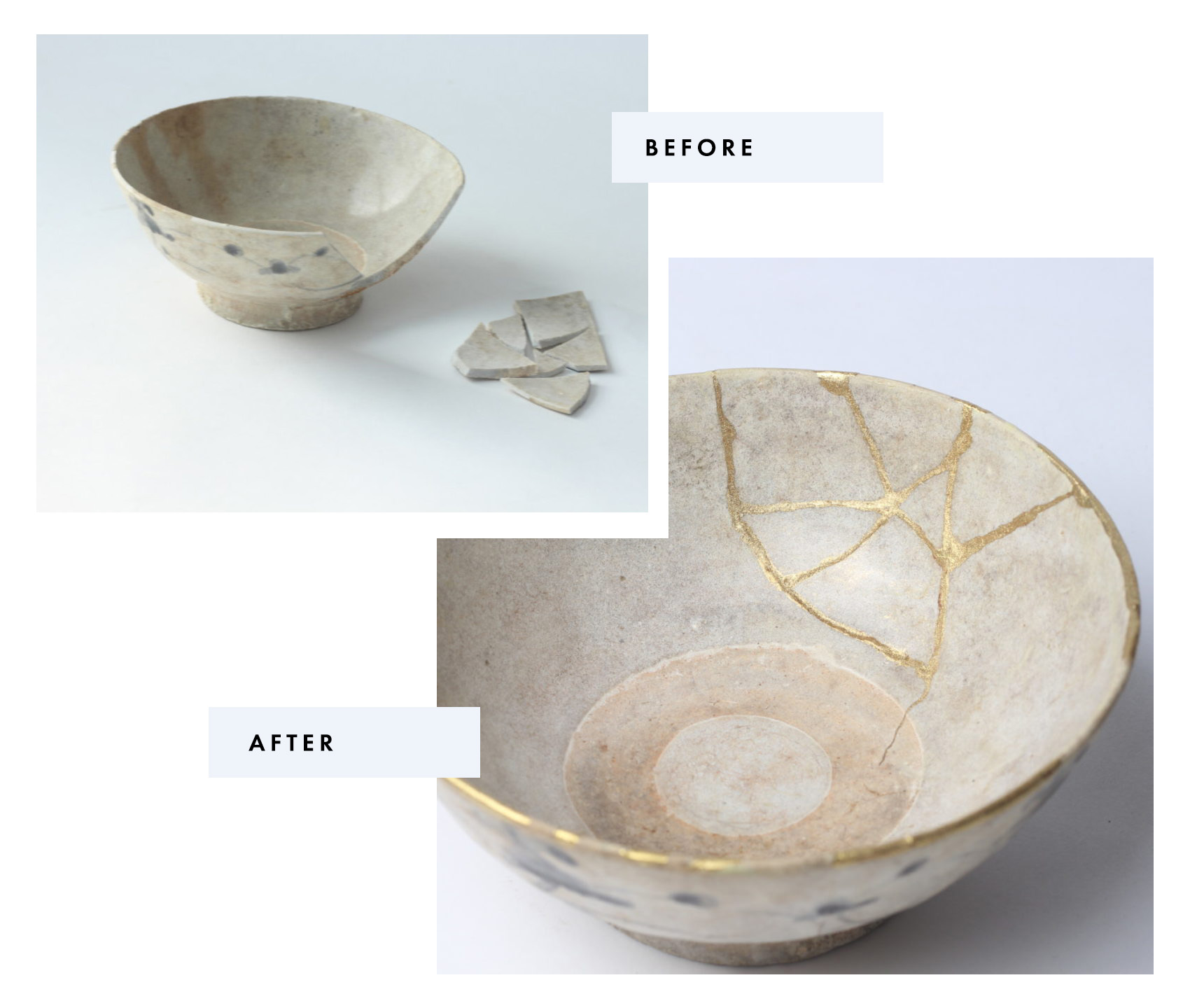The image consists of two photos labeled "before" and "after," positioned at the top left. The "before" photo, situated in the upper left corner, shows a small, stone or ceramic bowl with a dark gray, marble-like pattern featuring shades of light brown and black. A piece is missing from the side, and approximately six broken fragments are placed on a white surface next to the bowl. In contrast, the "after" photo, slightly larger and below the "before" photo, depicts the bowl fully restored. The broken pieces have been meticulously reassembled with a sparkling gold adhesive, which traces the cracks and forms an elegant gold inlay around the rim. This adhesive, possibly used for both structural and decorative purposes, adds a notable aesthetic element to the repaired bowl. The angle of the "after" image looks down into the bowl more from above, giving a better view of its repaired structure and the shimmering golden lines that now define its form.